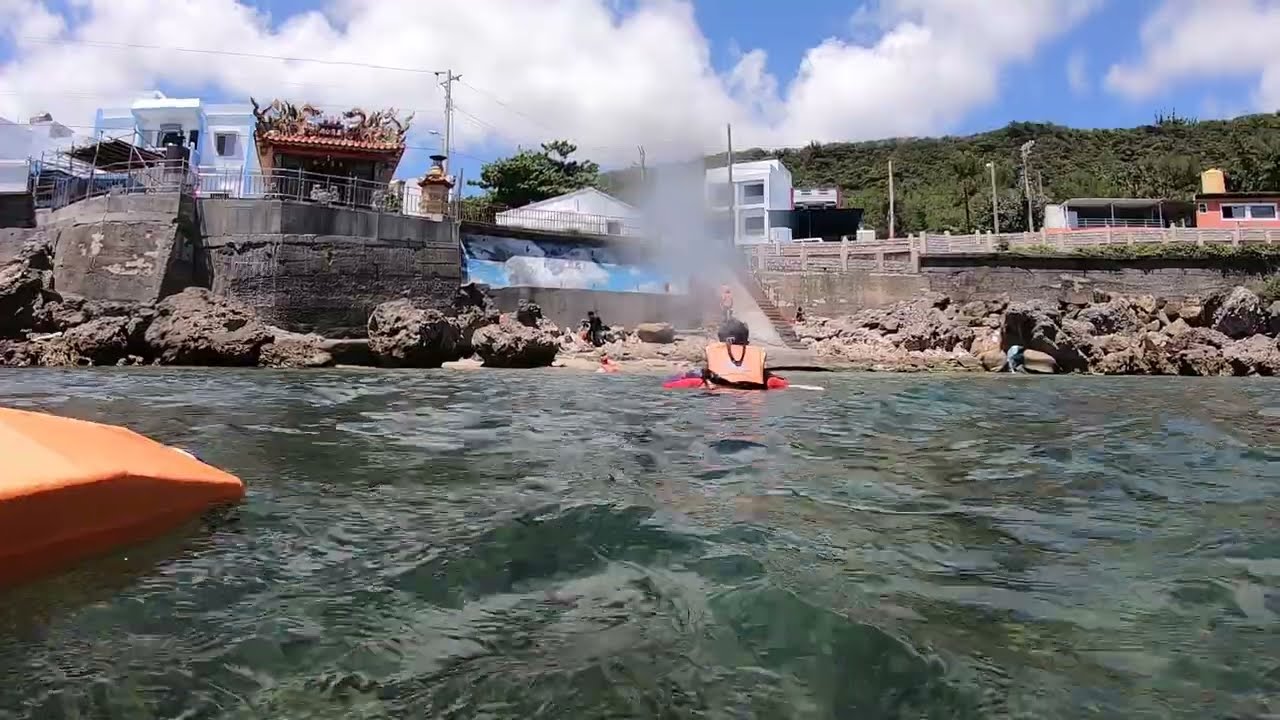In the photo taken from the perspective of someone in calm water, a boy wearing an orange life jacket and possibly black hair is seen holding onto a red flotation device. He appears to be swimming in a harbor filled with rocks, with the coast featuring a vertical wall and no sandy beach. The background showcases a small, possibly Grecian-like town built on a rocky coastline, with colorful buildings, including blue, white, and red structures, creating a picturesque scene. The sky is blue, dotted with numerous white clouds, indicating it's the middle of the day. On the shore, several people are present, with structures like houses, a possible restaurant, and greenery on a hill behind it. The image lens is slightly wet, resulting in a water drop partially obscuring the view but not diminishing the overall clarity of the scene. The overall setting suggests a serene and lively coastal environment.